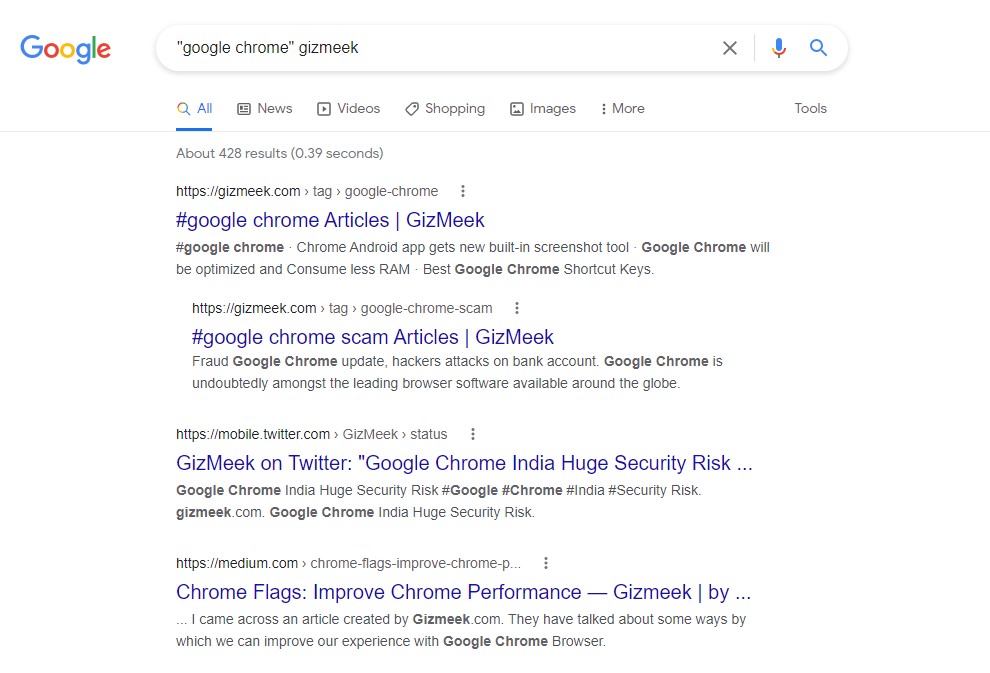The image displayed is a screenshot of a Google search results page, where the search query entered is "Google Chrome" combined with the term "gizmig" within quotes. The search results are generated under the "All" tab, totaling 428 results, delivered in a rapid 0.39 seconds. 

The first result is a link to HTTPS://gizmig.com, featuring several articles related to Google Chrome. One of these articles discusses general information about Google Chrome, while another explores potential scam issues associated with the browser, both hosted on the same website.

Further down the results page, another link directs to an article hosted on HTTPS://mobile.twitter.com, and yet another to a piece on HTTPS://medium.com. These entries all include the searched terms "Google Chrome" and "gizmig."

At the top-right corner of the search box, there is an 'X' icon, which users can click to clear the search query and start a new search. Additionally, next to the 'X' is a microphone icon, providing a feature for voice-activated searches. Lastly, there is the familiar search button that users can click to initiate the search after entering their text query.